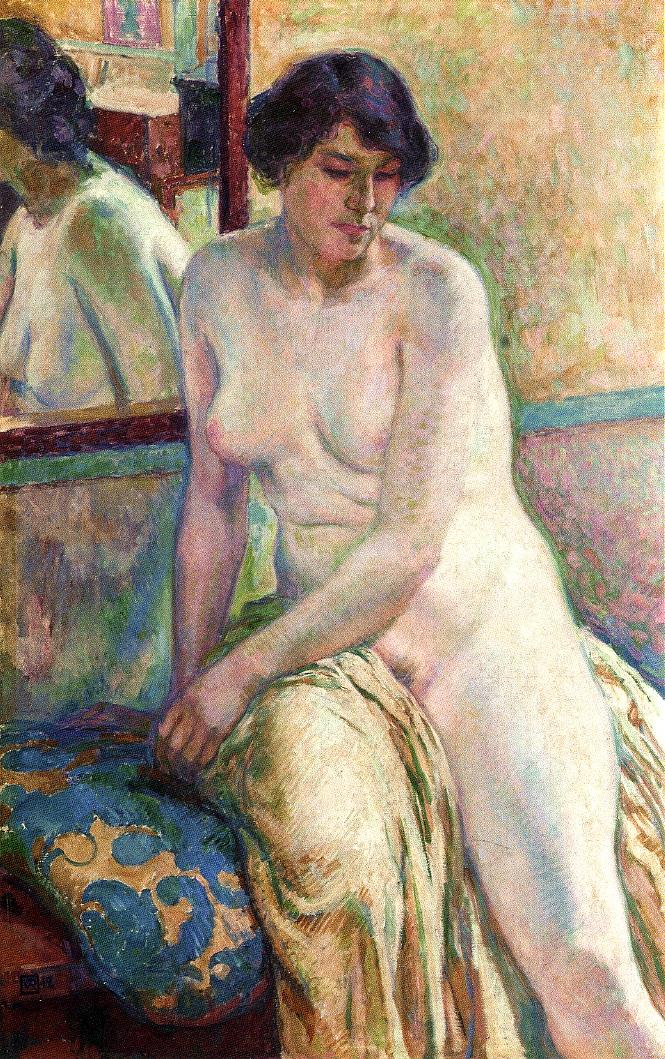The image is a vertically aligned rectangular painting depicting a partially nude woman with very light skin, sitting pensively on a wooden stool adorned with a blue pillow featuring a gold design. The woman has short to medium-length dark hair and gazes downwards towards the floor. Her right leg is modestly covered by a yellowish blanket, revealing her left leg entirely. A mirror behind her reflects her upper arm and chest, as well as a portion of a desk. The wall in the background has a brown textured appearance, adding depth to the scene along with a wooden frame around the mirror. The overall composition is detailed, capturing the reflective and somber mood of the moment.